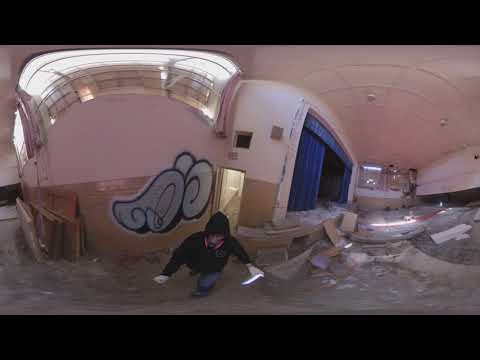The image showcases a distorted fisheye lens view inside a dilapidated, abandoned building, likely in the middle of the day. Dominating the scene is a man in a black hoodie and blue jeans, walking towards the camera from the center of the frame, with his face obscured by the hood. He appears to be a graffiti artist, as he is holding a spray can and standing in front of a wall adorned with gray graffiti. The floor beneath him and around the room is strewn with various trash and debris, adding to the rundown atmosphere. To his left (right side of the image), a large stage with a blue curtain is visible, contributing to the sense of neglect within the space. The setting is further characterized by a light pink rooftop and sunlight that filters in through a high, elevated window just beneath the ceiling, casting light onto the scene below.